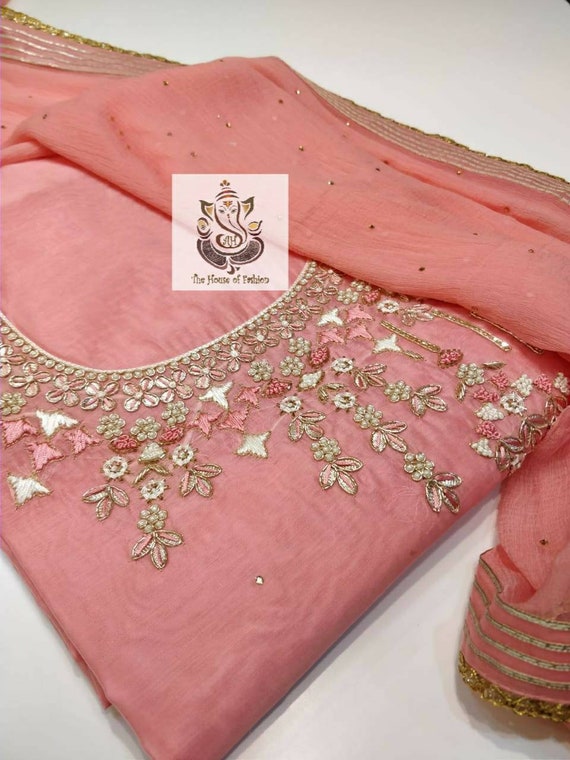This image showcases a beautifully ornate piece of clothing that appears to be an Indian top or dress. The main fabric is a delicate pale pink, adorned with intricate and vibrant embroidery. The needlework around the neckline features a combination of dark rose, various shades of pink, white, and gold thread, creating a richly detailed and attractive design. Additionally, gold trims enhance the elegant appearance of the garment, which includes possible sleeves or an accompanying scarf with similarly adorned edges.

The clothing item is carefully displayed on a flat surface. A label is partially visible and features a stylized elephant, potentially indicating the brand as "House of [name unclear]." The workmanship appears to be of high quality, with embellishments such as beading and bugle beads, as well as small gold details scattered throughout the fabric, further enhancing its luxurious appeal. The overall design and craftsmanship suggest that this piece is not only visually stunning but also finely made, likely to be associated with traditional Indian attire.